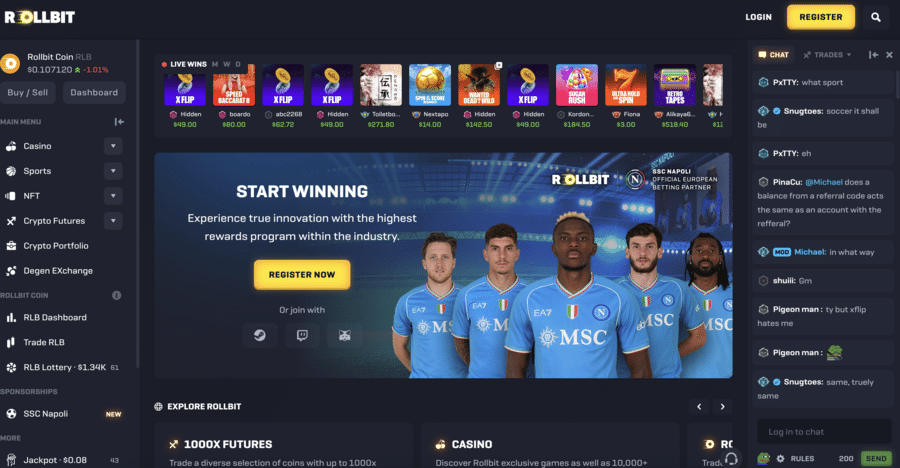This is a detailed screenshot captured from a computer screen showcasing a promotional banner for an online betting platform. The background is dark, creating a striking contrast with the content displayed. The left and right sides of the screen are mostly filled with text, highlighting various features of the platform. At the center of the image, there's a prominent picture featuring four young men dressed in soccer uniforms, standing against a blue backdrop.

Above these players, the text "ROLLBIT: BSC Napoli Official European Betting Partner" is prominently displayed. The upper left corner of the image features the platform's logo "Rollbit" and a "Rollbit coin number." Additionally, navigation options such as "Casino," "Sports," and "NFT" are listed, indicating different betting categories available on the site.

Just below these navigation options is a vibrant call-to-action section with a yellow button labeled "Register Now," inviting users to join and start betting. Another caption at the top left corner reads, "Start winning, experience true innovation with the highest reward program within the industry," emphasizing the platform's commitment to offering a rewarding betting experience.

Further enhancing the promotional feel, there is a bar above the soccer players' image that displays real-time information like "Live Wins" along with various icons. One icon features a golden soccer ball with the associated number “$14,” and another labeled “X Flip” shows animated coins flipping, indicating a value of "$49."

This comprehensive layout and vibrant presentation clearly aim to attract users to explore and participate in the various betting options offered by the platform.